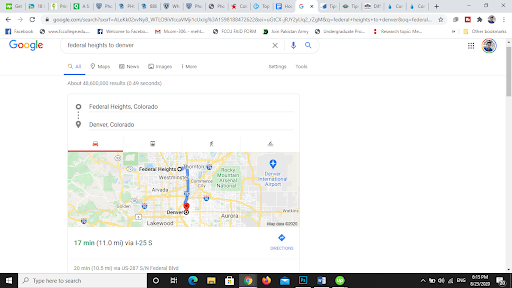This image depicts the Google Maps interface on a web browser, showcasing a route from Federal Heights, Colorado, to Denver, Colorado. The browser has approximately 15 tabs open along the top. In the upper left corner, the prominent Google logo is visible. The map highlights a blue line indicating the route between the two locations, suggesting a straightforward path. Below the map, a detailed description states that the journey covers 11 miles and takes about 17 minutes via I-25. A "Directions" button is also visible to the right, ready to offer additional navigation details.